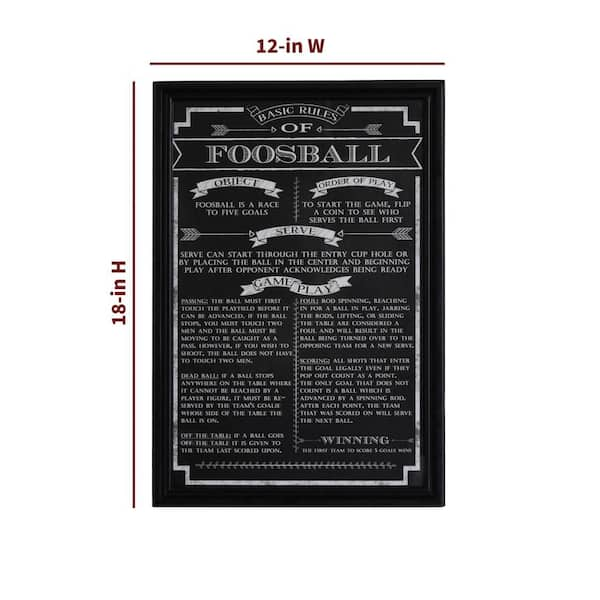This image features a black poster designed as a wall sign, framed in a matching black frame. The poster measures 12 inches in width and 18 inches in height. It is a guide titled "Basic Rules of Foosball," presented in white text on a black background. The layout is structured with sections delineated by little white banners, including the Object of the Game, Order of Play, Serve, and Gameplay. According to the poster, the objective of foosball is to be the first to score five goals. To determine the starting player, a coin toss is suggested. Players can begin the serve either through the entry cup hole or by placing the ball in the center after the opponent acknowledges readiness. Detailed rules for gameplay are also provided, highlighted with small arrows to guide the reader through the text.